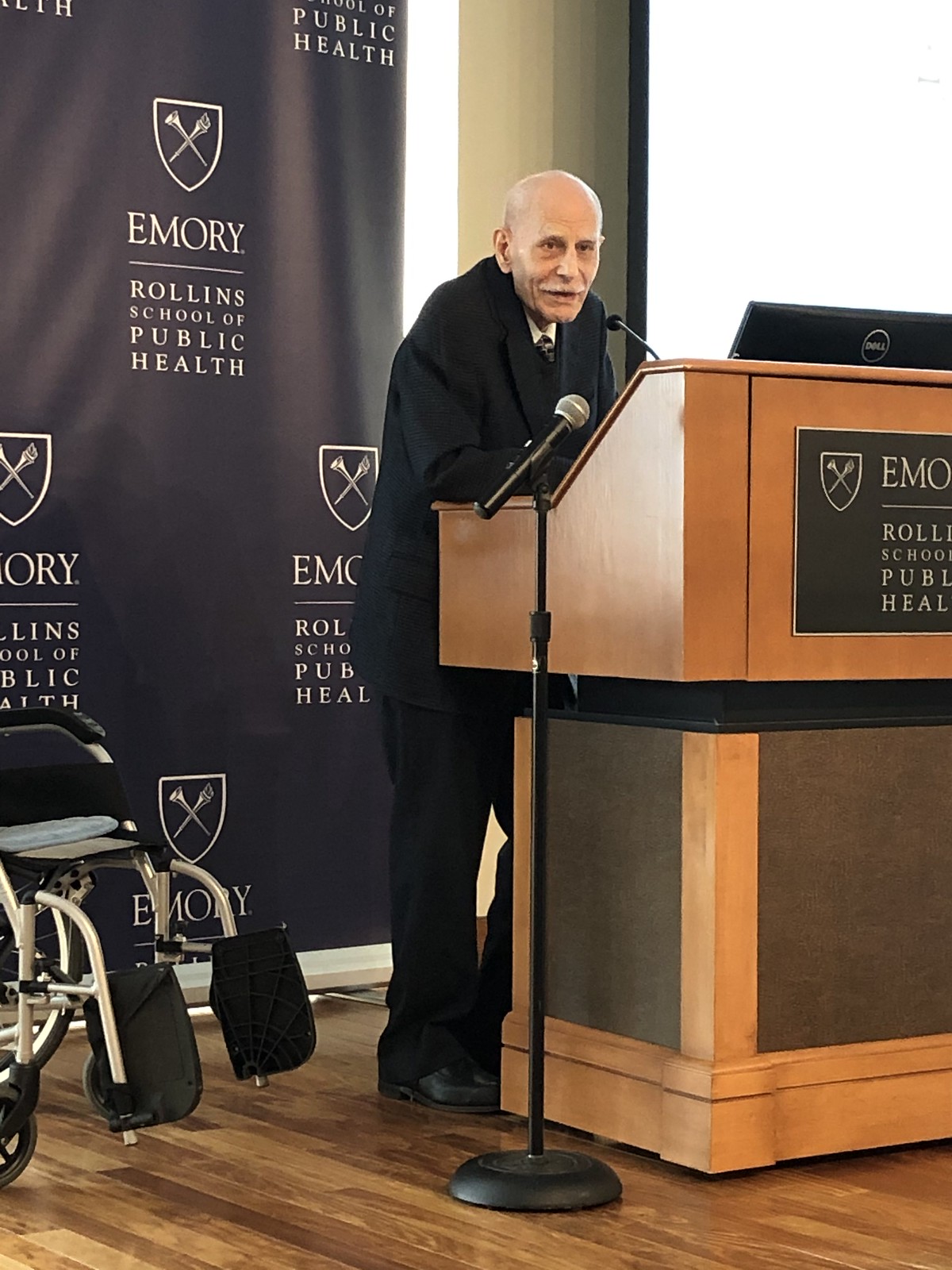In this photograph, an older gentleman, with a graying white mustache and mostly bald head, stands hunched over a wooden podium at the Emory Rollins School of Public Health. He is dressed in a black suit, black pants, black shoes, and a white button-down shirt with a tie. Positioned centrally in the image and facing the camera, he appears to be giving a presentation. The podium, situated center-right in the frame, features a plaque displaying part of the school's logo. A Dell computer and two microphones—a smaller one directly in front of him and a larger one to the left of the podium—are placed atop it.

Behind the speaker, a blue banner adorned multiple times with the Emory Rollins logo creates the backdrop. To his left, an empty black wheelchair suggests he recently rose from it. The background also includes the partial view of a white window on the right side. The photograph is set indoors, likely within an auditorium, given the professional environment and the arrangement of objects suggesting a formal event.